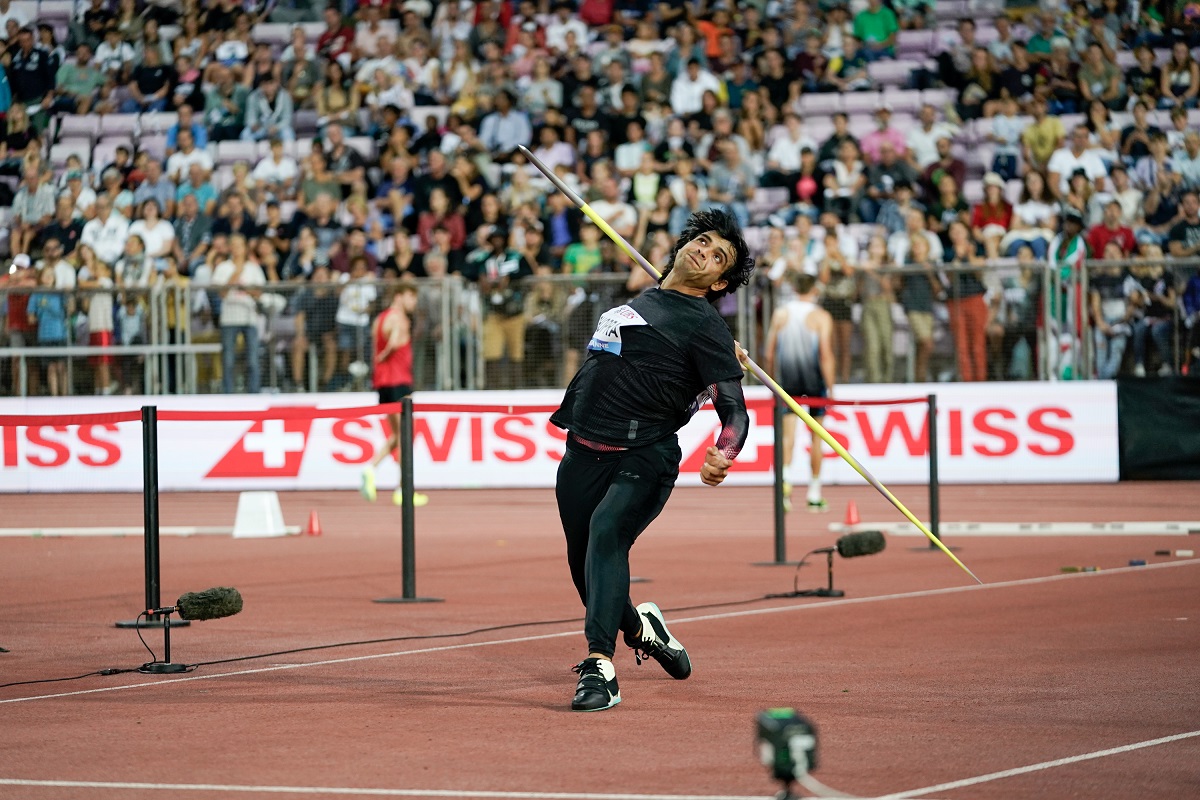In this dynamic action shot taken at a track meet, a female javelin thrower is captured mid-throw amidst the grandeur of a massive stadium filled with spectators. She is dressed in a sleek black athletic outfit, her right arm dramatically extended behind her holding a yellow javelin with a stainless steel tip. Her poised stance reflects the intensity of the moment; her left foot is firmly planted on the brown dirt track, while her right leg is slightly lifted, toe pointed towards the ground. Her short, curly black hair frames her face, contorted in a focused expression as she looks skyward.

The scene is set against a backdrop of a bustling crowd, their heads converging towards the center of the image to witness her performance. Just behind her, there is a prominent white banner displaying the red word "Swiss" repeatedly. Adding to the competitive atmosphere are four black poles with a red tape strung across them, serving as a barrier for the audience. This pulsating energy and detailed setup highlight the athletic prowess and determination of the javelin thrower as she competes.